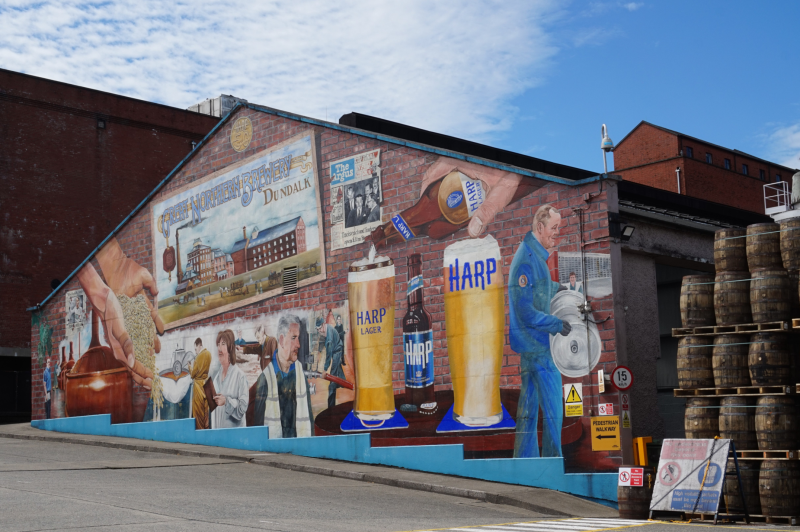The image depicts a vivid mural covering the side of a triangular-shaped, red brick building, possibly a brewery. The mural is filled with various beer-related illustrations, prominently featuring the brand 'Harp' in blue text. Central to the artwork is a depiction of hands pouring beer into large glasses from a Harp bottle, with additional Harp bottles and glasses spread throughout the scene. On the right side of the mural, a man in a blue suit is shown carrying a beer keg. To the left, a pair of hands are seen holding and spilling hops or grain next to a brown basket. The background includes various people in different work attire, likely representing brewery workers, with a woman holding papers and workers in the distance. Further left, another segment of the mural showcases a brewery building labeled "Northern Brewery Dundalk." Real elements blend into the scene with an actual stack of barrels positioned next to the brick building, along with red buildings and a blue sky filled with clouds in the far background.